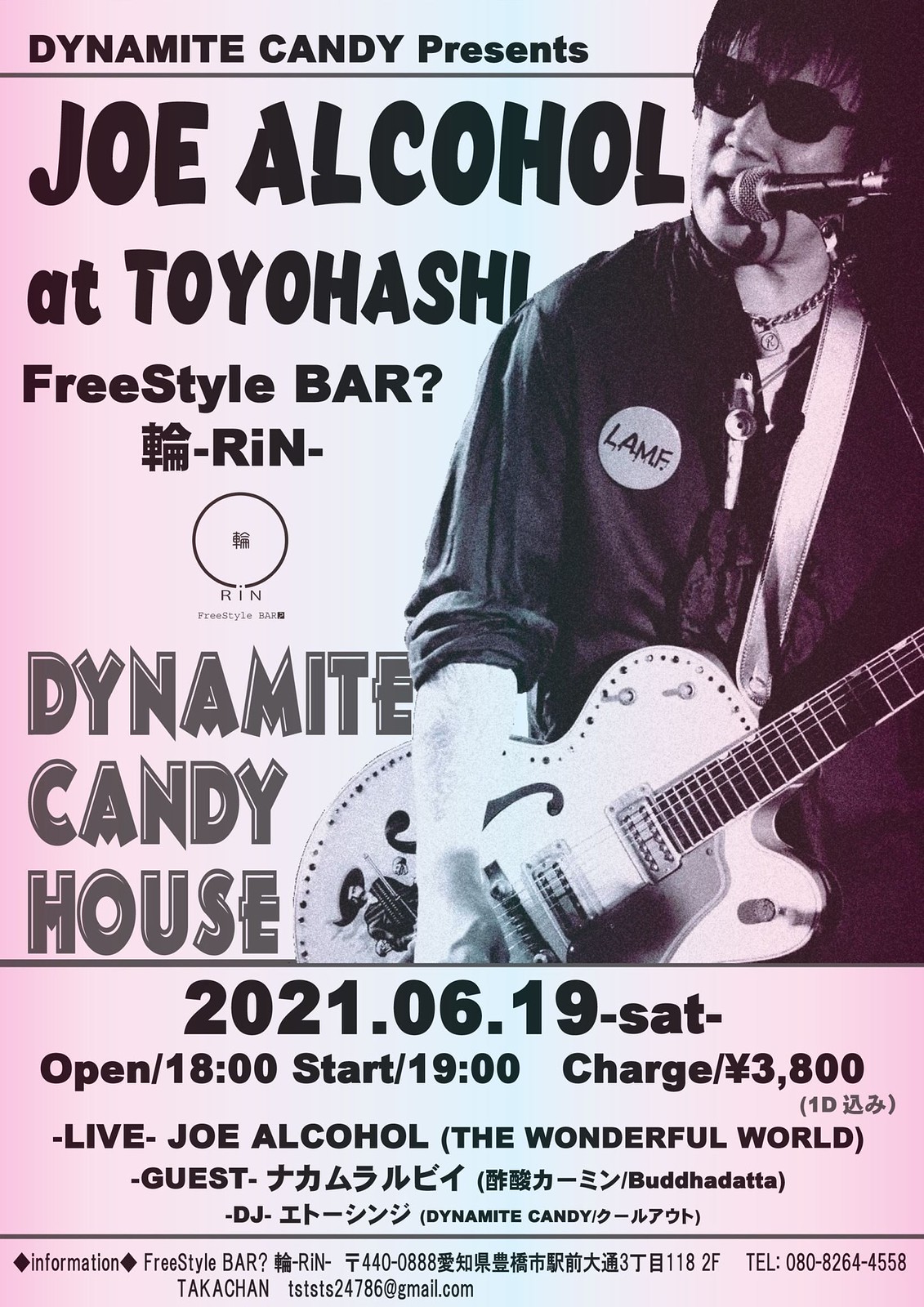This color photograph is an advertising flyer with a cotton candy-colored background, featuring light pink on the sides and a hint of light blue fading through the center. Dominating the right side is a black and white photo of a singer, identified as Joe Alcohol. He has shaggy hair with bangs, and is wearing black sunglasses. He is passionately singing into a microphone while holding a guitar, dressed in a black shirt adorned with silver necklaces and a round white badge with the text "LAMF." To the left, the flyer is adorned with several lines of text. At the top, in black text, it reads "Dynamite Candy Presents Joe Alcohol at Toyohashi Freestyle Bar?" Below that, in smaller gray text, it says "Dynamite Candy House." The bottom section lists details including the date, "2021-06-19, SAT," with the times "open 1800, start 1900," and the entry fee "Charge 3,800 yen." Additional performance details, addresses, and phone numbers are listed, some in an East Asian language.